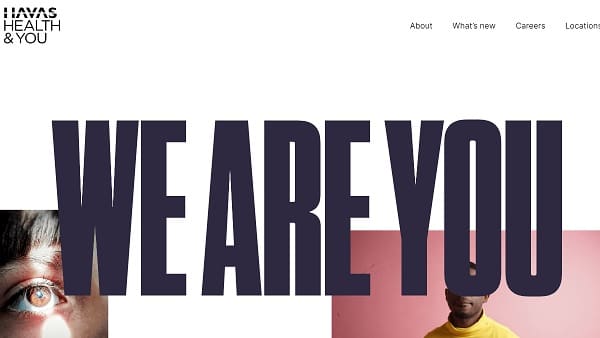Here is a more detailed and cleaned-up caption for the described image:

---

This image captures the top banner area of a webpage belonging to HAVAS Health NU. In the upper right-hand corner, the logo "HAVAS" is prominently displayed in capital letters. A distinctive white line runs horizontally through the middle of the logo, creating an effect as if the bar of the "H" has been erased and continuing this line through the rest of the letters.

At the top left of the page, the navigation menu is listed in a standard black font, featuring the options "About," "What's New," "Careers," and "Locations." 

Below the navigation bar, the main header section of the webpage displays the phrase "WE ARE YOU" in large, bold, black capital letters against a white background. 

Embedded within this header are two photographs partially visible beneath the text. To the lower left, there is a close-up image of a person's face, showcasing a brown eye, an eyebrow, and a portion of bangs. This individual appears to be white, though it's unclear if the person is male or female.

On the right side, another person is partially visible. This appears to be an African-American male wearing a yellow turtleneck. His lips, part of his ears, and a small portion of his face are visible through the "O" in the word "YOU," set against a pink background.

---

This caption offers a detailed and clear description of the webpage's top section, its design elements, and embedded imagery.